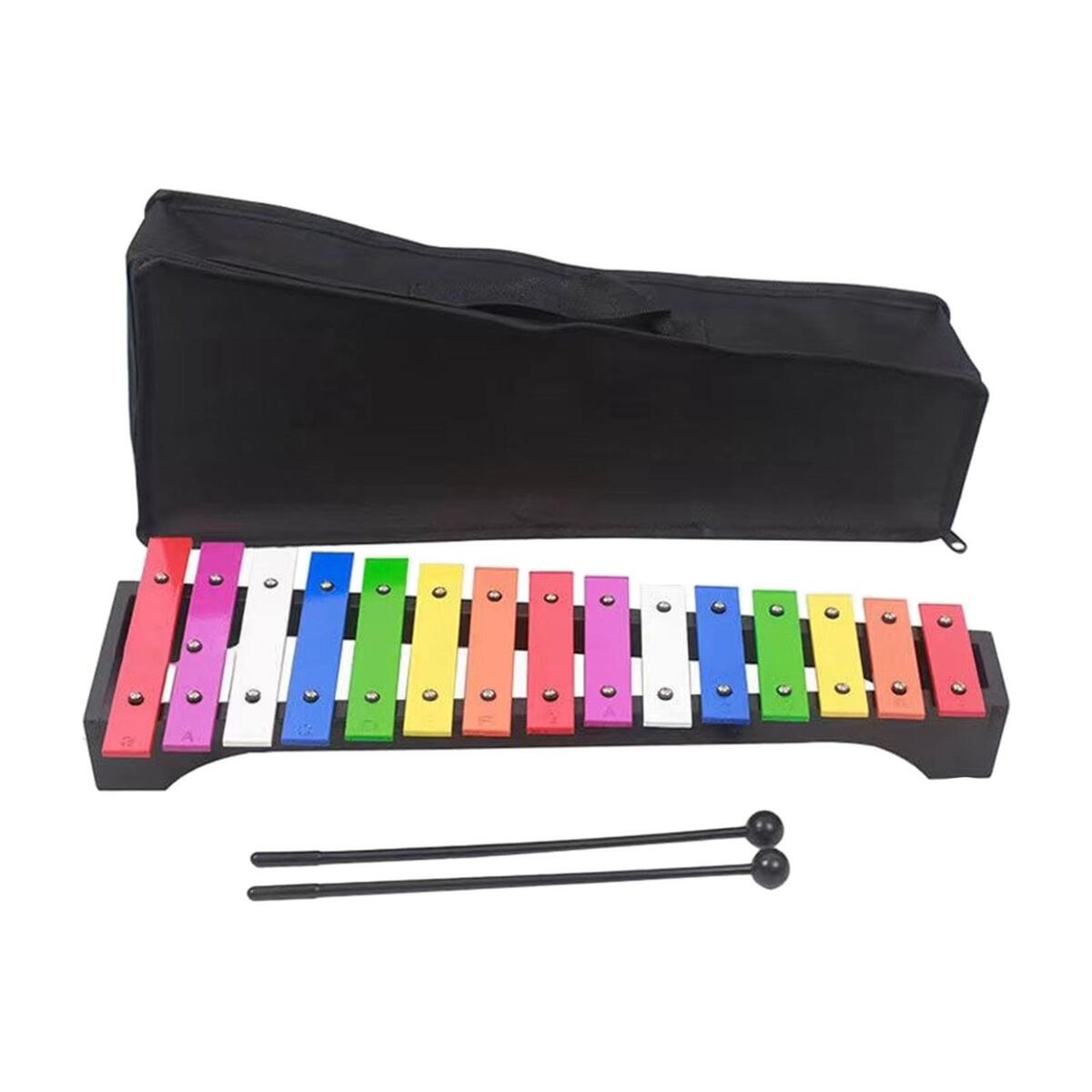This is a product image from a music supply catalog featuring a brightly colored xylophone, displayed on a plain white background. The xylophone is centered in the image, with larger keys on the left and smaller ones on the right, and features approximately 15 to 20 keys. The keys come in an array of colors including red, purple, white, blue, green, yellow, and orange, arranged in a non-repeating pattern. The xylophone is mounted on a sleek black base that tapers from larger on the left to smaller on the right. In front of the xylophone, there are two identically shaped black mallets with spherical tips for striking the keys. Behind the xylophone, there is a black zip-up soft-sided case, trapezoidal in shape to match the xylophone’s tapered design, with a fabric handle on top for easy carrying.